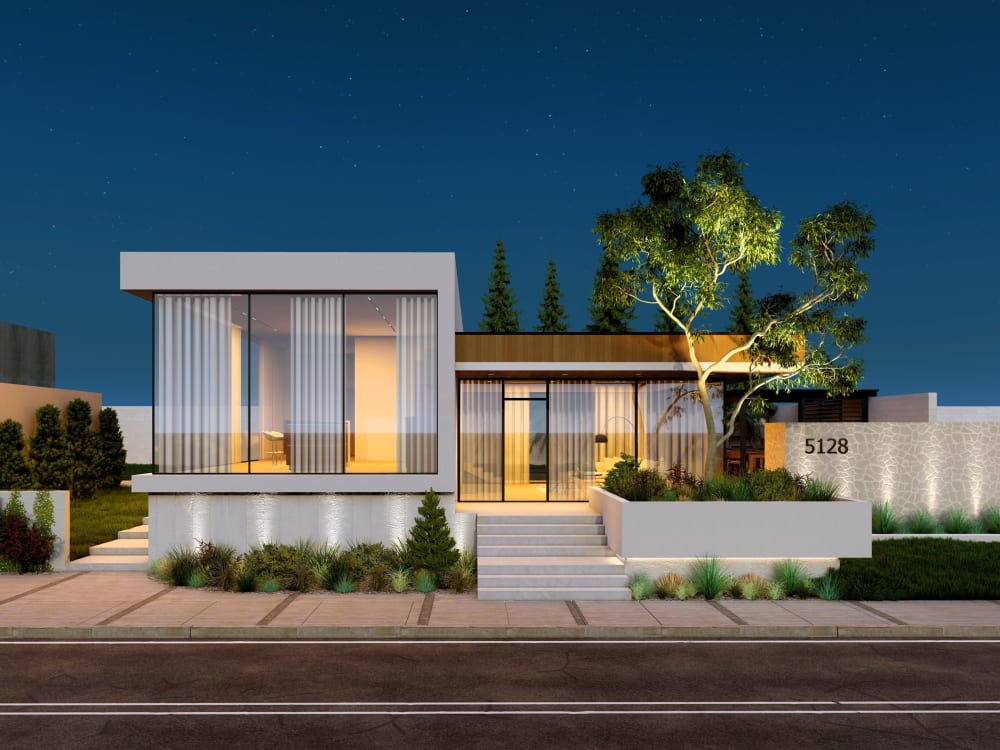This image showcases a strikingly modern and luxurious rectangular house, predominantly constructed from glass, exuding an almost digitally designed aesthetic. The house, marked with the number 5128 on a brick stone wall, is painted white with wooden accents at the top. Massive floor-to-ceiling windows adorned with thin curtains offer glimpses of the minimally furnished interior bathed in warm yellow lighting. The house is set against a clear, deep blue night sky sprinkled with stars, highlighting the illuminated structure. A prominent staircase leads up to the entrance, flanked by greenery, including a large tree in the front yard and additional smaller trees on the left and behind the house. The scene features a beige sidewalk and a dark brown road with distinct white lines running down the middle, emphasizing the house's contemporary elegance amidst its natural surroundings.